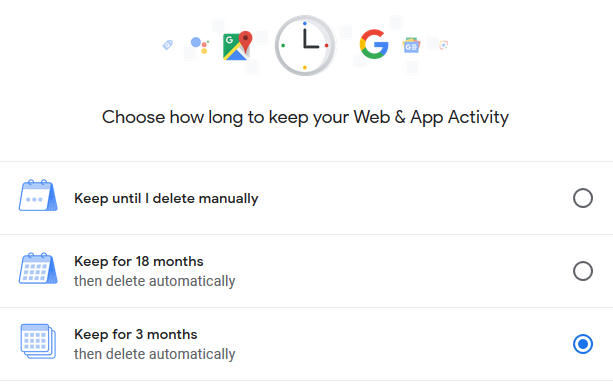On a white background, the illustration features a central cartoony clock with a gray outline frame and a white face. The clock displays black hands set at 3:00, with colored dots marking the hours: blue at 12, red at 3, yellow at 6, and green at 9. To the left of the clock, a series of icons illustrates various Google services. 

From left to right, the sequence starts with a clothing tag bearing a "G", followed by icons for Google AI, Google Maps, the central clock, the Google multi-colored "G", a likely icon for Google Documents, and an unidentified icon. Below these icons, in black text, is the instruction: "Choose how long to keep your web and app activity."

Underneath the text, a gray line divides three options:
1. "Keep until I delete manually" - with an empty circle on the right.
2. "Keep for 18 months then delete automatically" - with an empty circle on the right.
3. "Keep for 3 months then delete automatically" - with a blue check-marked circle on the right.

Each option is preceded by distinct, blue calendar icons.